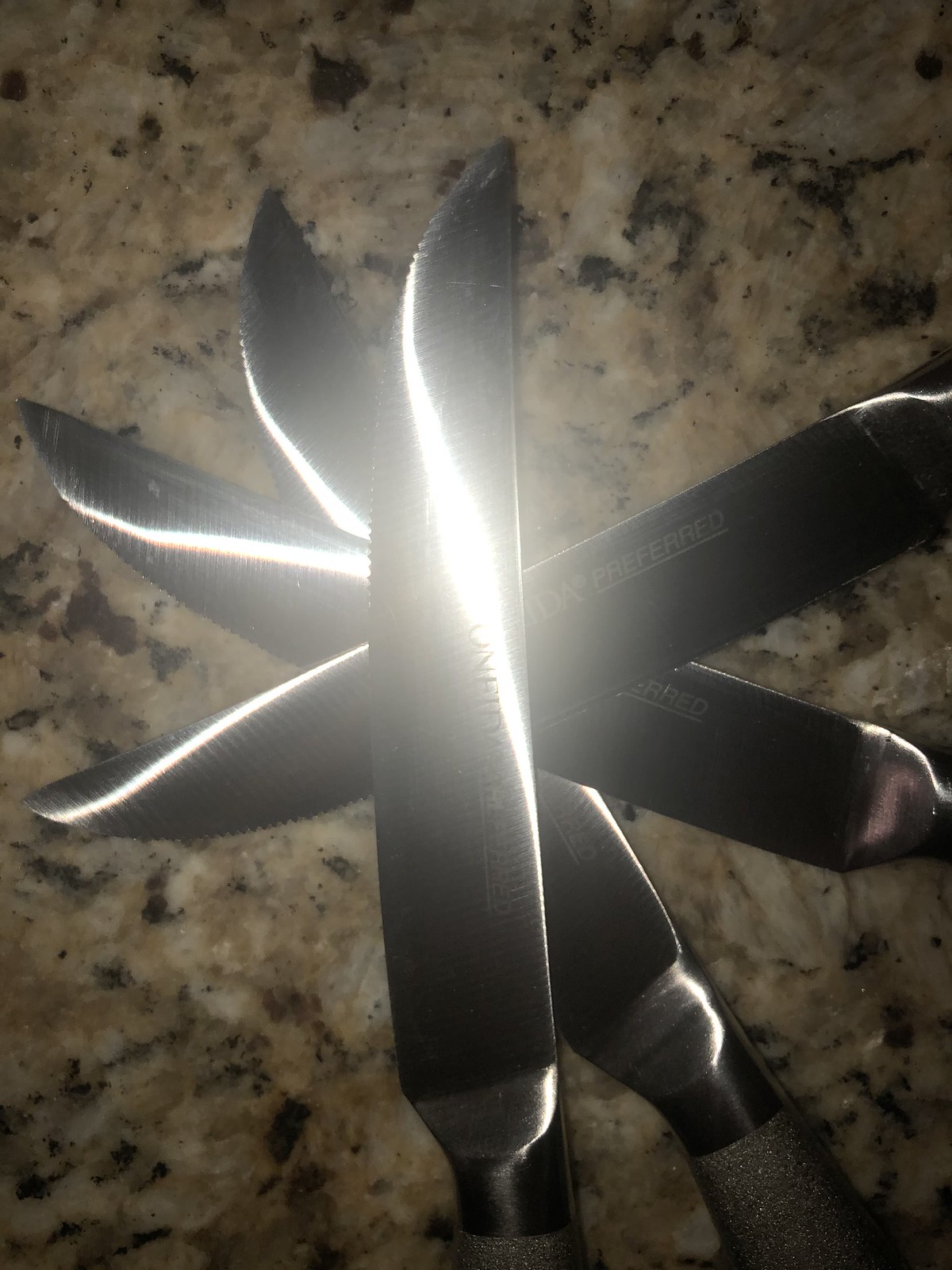This image captures a close-up view of four silver butterknives meticulously arranged in a star-like pattern on a tan granite countertop with specks of chocolate brown and black. The knives, about eight inches long, feature slightly serrated blades and are artistically fanned out, with their points directed towards the upper left of the frame. A direct light source from above casts bright, integral sign-shaped reflections down the center of each knife, highlighting the word "Preferred," which is underlined in white on the blades. The handles, adorned with gray sparkles, are also visible, adding to the overall aesthetic. The precise arrangement and intense white reflections from the light create an abstract visual effect that draws immediate attention.